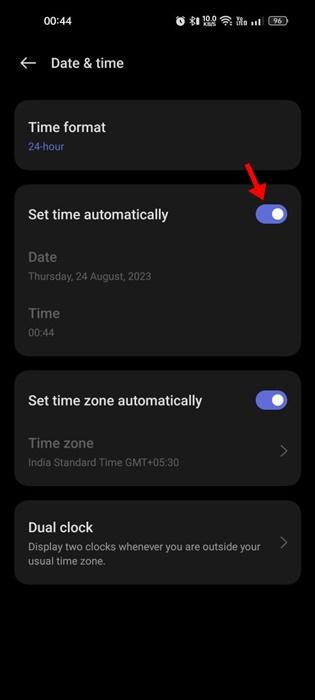The image displays the date and time settings screen on a cell phone. At the top left corner, there is a back arrow pointing to the left. To the right of this arrow, "Date and Time" is prominently displayed in white font. Below this heading, the screen is divided into four distinct sections separated by light gray blocks, which contrast with the darker gray background of the settings page. 

The first section is labeled "Time Format" in white font, and underneath this label, "24-hour: 09:00" is shown in blue text. The second section is titled "Set time automatically," featuring a blue toggle switch with a white button that indicates the setting is enabled. A red arrow points to this active toggle switch. The third section, "Set time zone automatically," also contains a similar blue toggle switch with a white button, showing this setting is enabled as well.